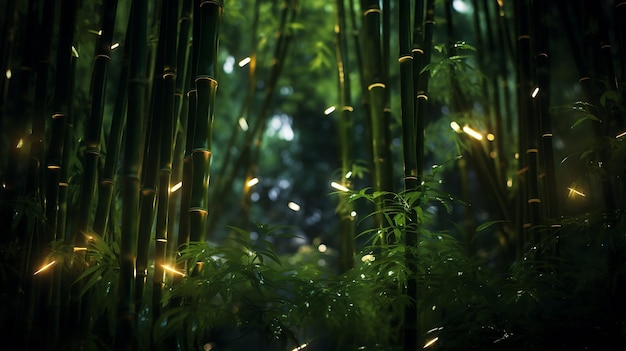This image depicts a vibrant bamboo forest captured from a low vantage point, giving a sense of immersion into this natural setting. The bamboo trees, characterized by their bright to neon green hues, densely populate the scene, creating an almost tunnel-like effect with their towering, slender forms. Sunlight filters through the branches, casting natural highlights and illuminating the vibrant greenery, with rays seemingly crashing into the forest and creating a dynamic interplay of light and shadow. The ground is covered in thick foliage, comprised of blades of grass and leaves, contributing to the dense, lush atmosphere. In the middle of the forest, there's a hint of blue light peeking through, potentially suggesting a clearing or an opening, adding depth to the perspective. Scattered throughout the image are small yellow specks, which look like floating particles, enhancing the ethereal feel of the scene. The overall effect is a vivid portrayal of a dense, sunlit bamboo forest with intricate lighting and rich colors melding into a serene yet lively natural tableau.